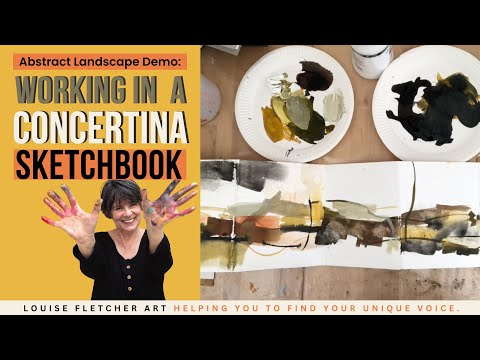The image shows the cover of a workbook or workshop guide on the left side, which has a yellow background and several prominent text elements. At the top of the cover, in black font on an orange banner, it reads, "Abstract Landscape Demo;" followed by "WORKING IN A" in green, all capitals, and "CONCERTINA" in white, all capitals. Below these titles, there is another orange banner with the word "SKETCHBOOK" in black, all capitals. Beneath this text, there is a picture of a Caucasian woman with short brown hair, smiling, and wearing a black shirt. She has paint smudges on the palms of her hands, indicating she has been finger-painting. At the very bottom of the cover, there is a white banner that says, "Louise Fletcher Art, helping you to find your unique voice" in black letters. To the right of the workbook cover, there is a wooden surface displaying two plates covered with various paints and a long strip of white paper featuring abstract watercolor art in orangish, grayish, and brownish tones.